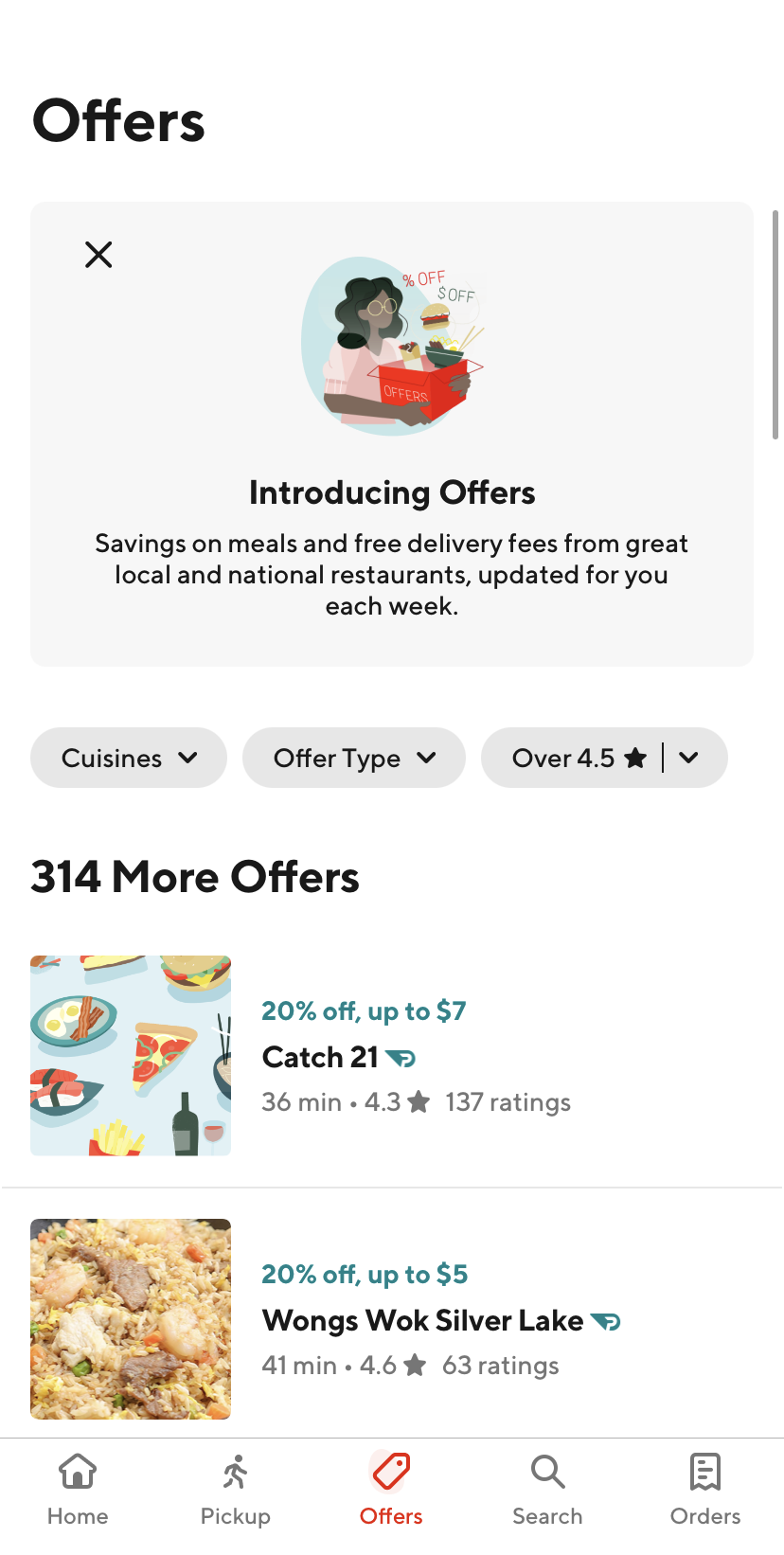The image appears to be a screenshot from a mobile application displaying meal offers. The top section features a white background with the word "Offers" prominently displayed in the upper left corner. Directly below, there's a gray box with an 'X' in the upper left corner for closing the window. Inside this box, an image of an African-American female, possibly holding a red container filled with food, is shown.

Beneath the image, the text reads: "Introducing Offers: Savings on meals and free delivery fees from great local and national restaurants updated for you each week". Below this introductory message, there are three drop-down buttons labeled "Cuisines," "Offer Type," and "Over 4.5 Stars."

Following these options, a heading states "314 more offers." The first listed offer showcases an image featuring various foods including a wine bottle and sushi. It promotes "Catch 21" with a discount of 20% off up to $7. The details include a delivery time of 36 minutes, a rating of 4.3 stars, and 127 ratings.

The second offer includes an image resembling fried rice with pieces of chicken and beef. It advertises "Wong's Walk Silver Lake" with a 20% discount up to $5, a delivery time of 41 minutes, a rating of 4.6 stars, and 63 ratings.